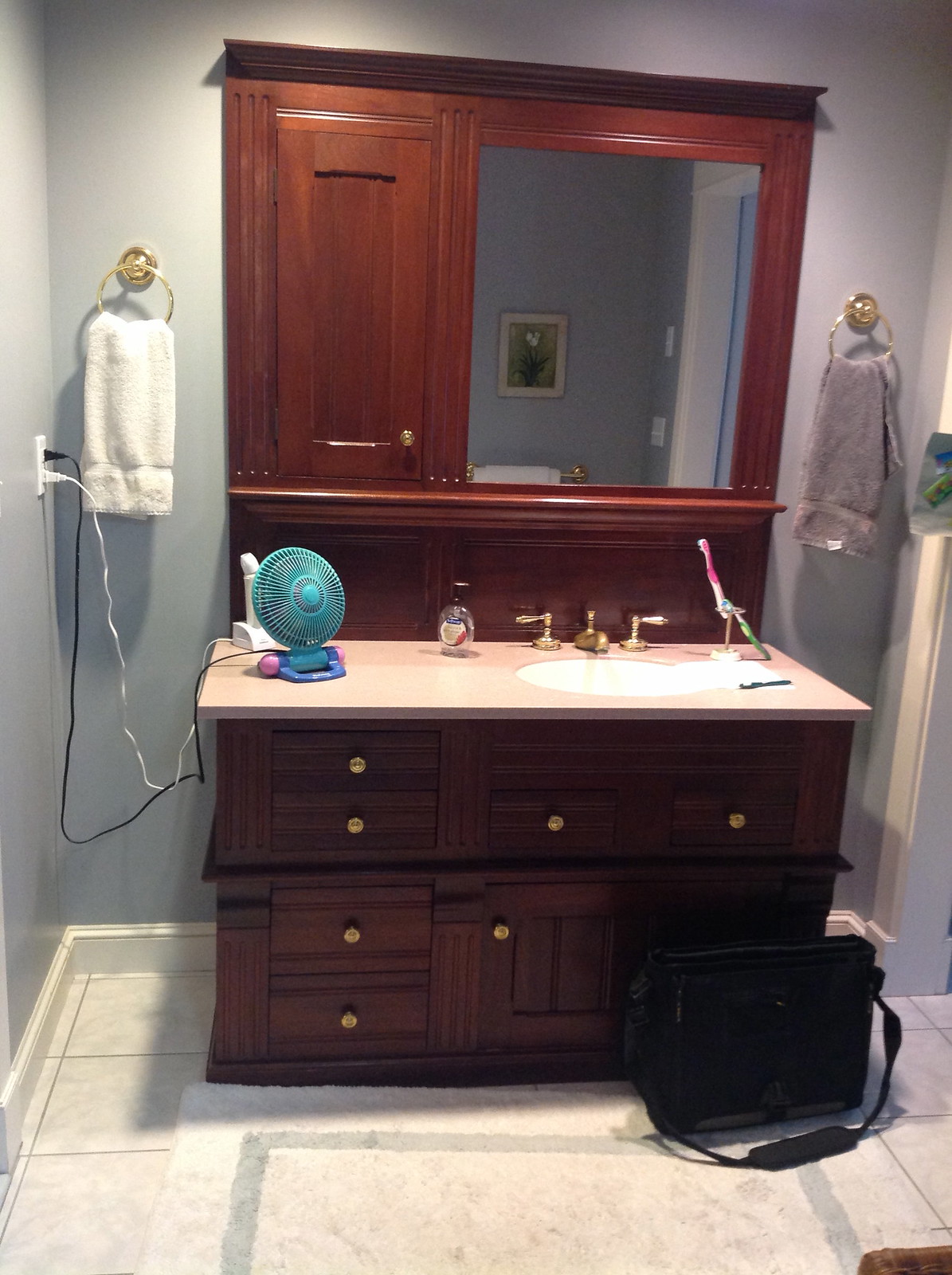The image captures a charming bathroom scene centered around a vintage-style wooden vanity. The vanity boasts a luxurious marble countertop, which features a pristine white sink adorned with elegant gold faucets and handles. Above the vanity, a large mirror reflects the softly illuminated space, hinting at overhead lighting.

Flanking the mirror are towel holders, each bearing a towel—one white on the left, and one gray on the right. Adding a touch of modern convenience, a small turquoise blue fan sits on the countertop, alongside essential items such as a hand soap dispenser and a toothbrush holder with a toothbrush.

On the tiled floor, a black laptop bag rests beside a fluffy white carpet, introducing a subtle contrast to the room’s grayish walls. To the right, the doorway with its white frame is partially visible, contributing to the overall airy and clean aesthetic of the space.